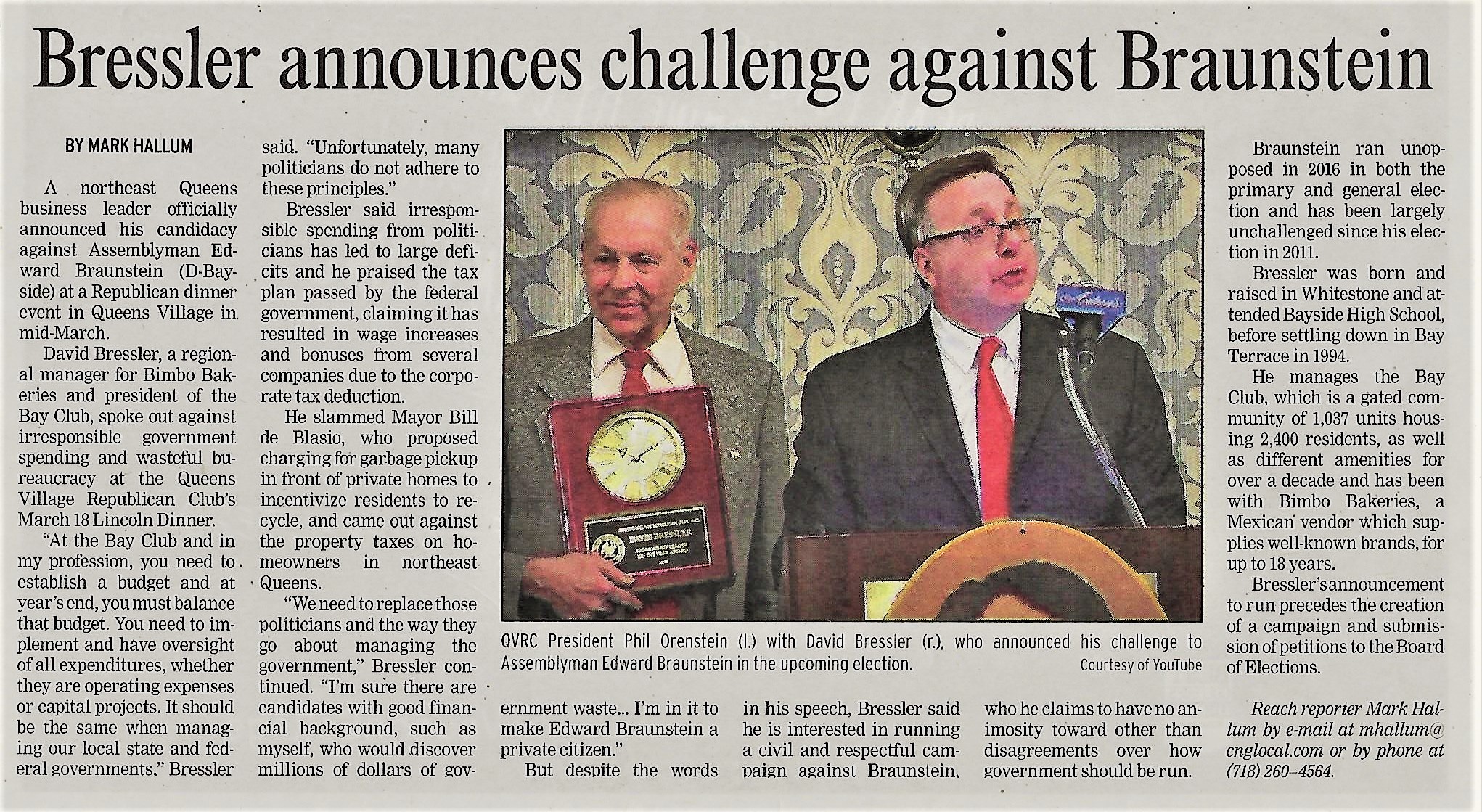Here's a cleaned-up and detailed caption for the described image:

---
A newspaper clipping features an article headlined "David Bresler Announces Challenge Against Braunstein." The article is printed on a grey background with black text and spans across six columns. At the center, a photo showcases two middle-aged men. On the left, a man with receding blonde hair is seen, while on the right stands a man in a darker grey, almost black jacket, a white shirt, and a red tie. He is holding a gold round clock mounted in a rectangular wooden frame, adorned with a black and gold plaque bearing tiny inscriptions. This man is identified as QVRC President Phil Olmstein, standing before a microphone. Behind him, the backdrop features an old-fashioned scrolling grey and white wallpaper design. The man on the left, David Bresler (indicated with brackets containing "C"), is challenging Assemblyman Edward Braunstein in the upcoming election. The article, written by Mark Hallam, starts by detailing Bresler's announcement at a Republican dinner event in Queens Village in mid-March. The detailed contact information for the reporter is partially obscured but mentions an email address and phone number. The image was sourced from YouTube, linking the print to digital media.